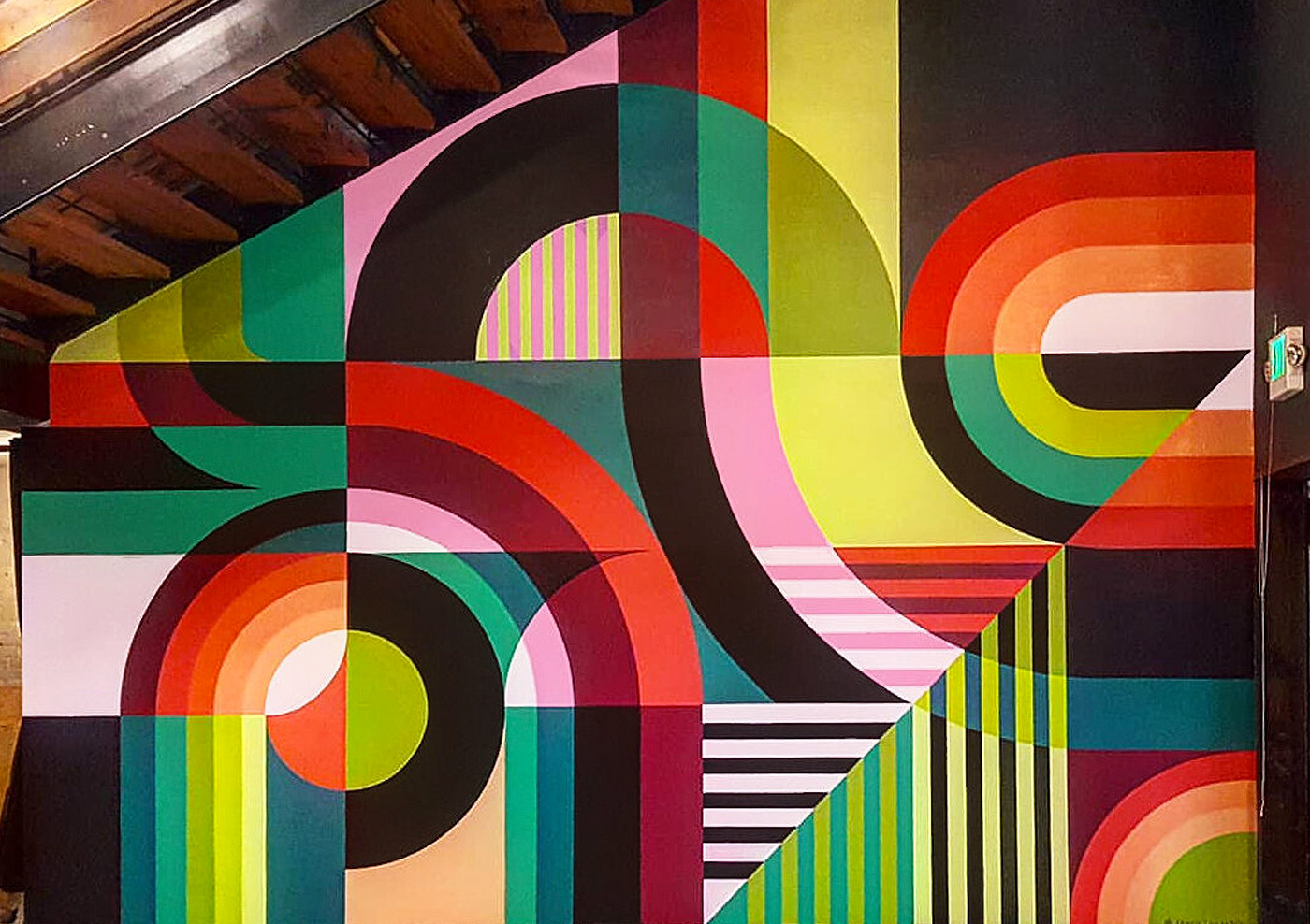This image captures a vibrant and eclectic wall mural bursting with an array of shapes and colors. Dominated by swirling curves, striking lines, and geometric forms, the artwork features a kaleidoscope of hues including bright pinks, reds, oranges, greens, blues, and browns. The left side of the mural is highlighted by an attic staircase in dark brown with black side bars, neatly nestled in the top left corner, while a wall-mounted fan control with a blue screen occupies the lower right. On the right side, a complex pattern resembling a racetrack weaves through the mural with bands of red, orange, light orange, and white curving gracefully. Beneath a prominent horizontal line, the colors cascade through a gradient of greens and blacks, finally reverting to a striking sequence of white, orange, and red. The mural, likely photographed indoors and head-on from a standing position, features no text but captivates through its dynamic array of shapes and vivid colors, coming together to create a mesmerizing piece of modern artwork.